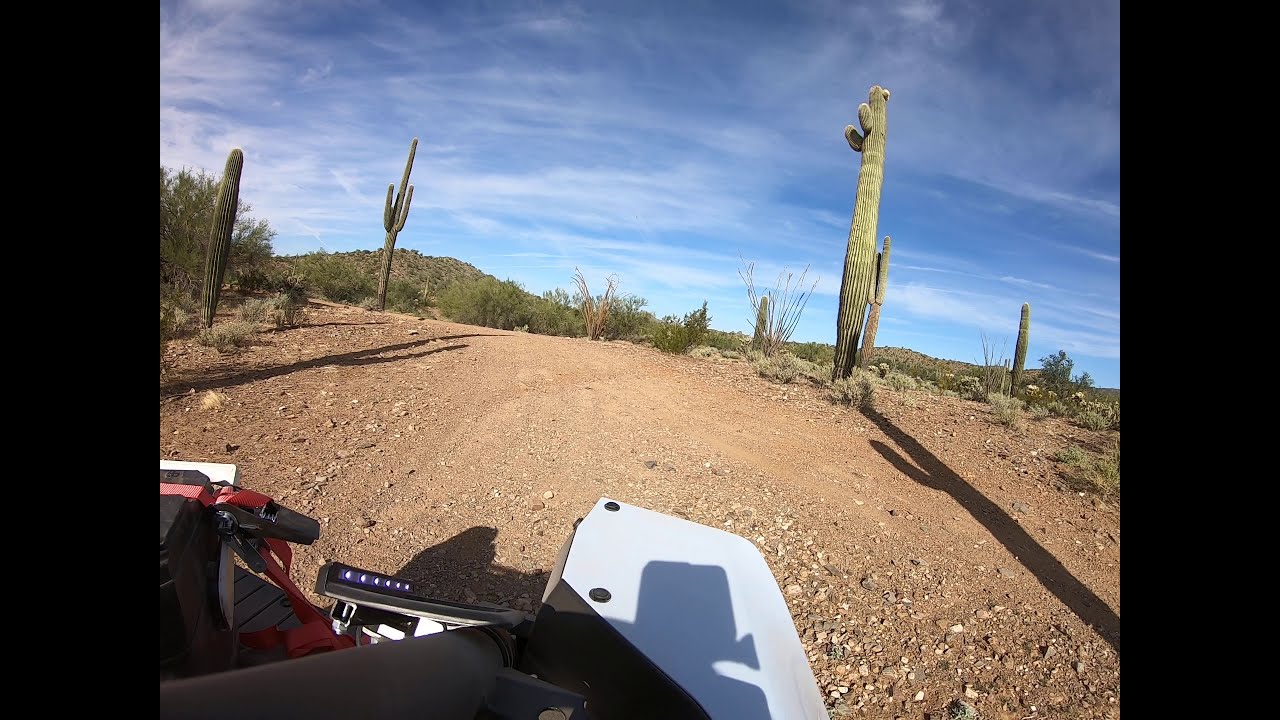This image is a detailed exterior color daylight photograph of a dry, dusty desert scene, framed by vertical black bars on the left and right. The photograph appears to be taken from the perspective of someone riding an ATV or a similar off-road vehicle, which is partially visible at the bottom of the image with elements featuring white, black, and red colors. The ground consists of a light brown dirt road littered with small rocks and gravel, showing tracks from previous vehicles. Scattered across the scene are tall, cylindrical green cactuses and smaller green shrubs, lending some color to the otherwise arid landscape. In the background on the upper left, there's a hilly area with sparse pale green vegetation. The sky above is a light blue, adorned with plenty of wispy, white clouds, which contrast beautifully with the overall desolate theme of the desert. The scene is further enriched with some low trees sprinkled throughout the area, adding to the sparse yet resilient plant life typical of desert environments.